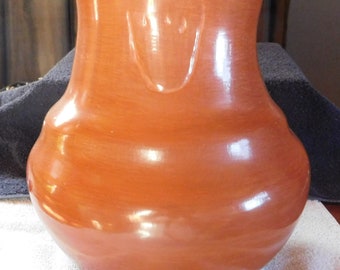The image features an orange, vase-shaped piece that appears to be made of glass or plastic. This object has a noticeable glare reflecting off its surface, suggesting it might be some kind of blown glass. It is seated on a small white platform, possibly a towel, placed on a table. Adjacent to this setup is another table draped with a gray cloth. The background includes walls on the left and upper right, which are a shade of gray. There also seems to be a bed or couch nearby, with a gray and black blanket casually strewn over it. The scene is lit in such a way that there is a pronounced white light illuminating the orange vase-like object, potentially giving off the appearance of a liquid or caramel texture due to the shine and reflections.